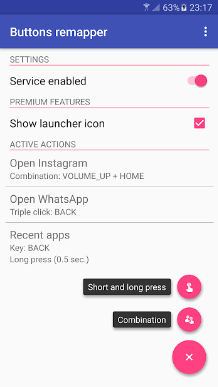The image displayed on a mobile screen shows an application interface with a blue top bar featuring a battery icon on the right side indicating 63% charge. To the right of the battery icon, the current time is displayed as 23:17. Beneath the top bar are three white circles aligned horizontally.

On the left-hand side of the main interface is the title "Buttons Remapper" in capitalized initial letters. Directly below, there is a section with a white background and the words "SETTINGS" written in all caps in bold black text. Under "SETTINGS," a thin hot pink line stretches horizontally across.

Following this line, in black text, the words "Service Enabled" and "Premium Features" are written. Adjacent to this, two circles are displayed: a larger hot pink circle on the right and a smaller light pink circle. A thin pink line cuts across this section.

Further down, black text reads "Show Launcher Icon" and "Active Actions," followed by a pink square with a white check mark inside. Another pink line extends horizontally across beneath this point. The text "Open Instagram" is followed by "Combinations: volume_up + home," presented in black.

A thin gray line separates the sections, below which the text "Open WhatsApp" can be seen, followed by "triple click: back." Directly beneath, another horizontal line appears. The text "Recent Apps: key back, back, back, long press (0.5 seconds)" is listed below in black. Completing this section are two white rectangles with gray borders; the first reads "short and long press" and the second reads "combination."

At the bottom of the image, there are three pink circles. The middle circle contains an "X," while the adjacent circles, from left to right, depict two fingers and one finger, respectively.